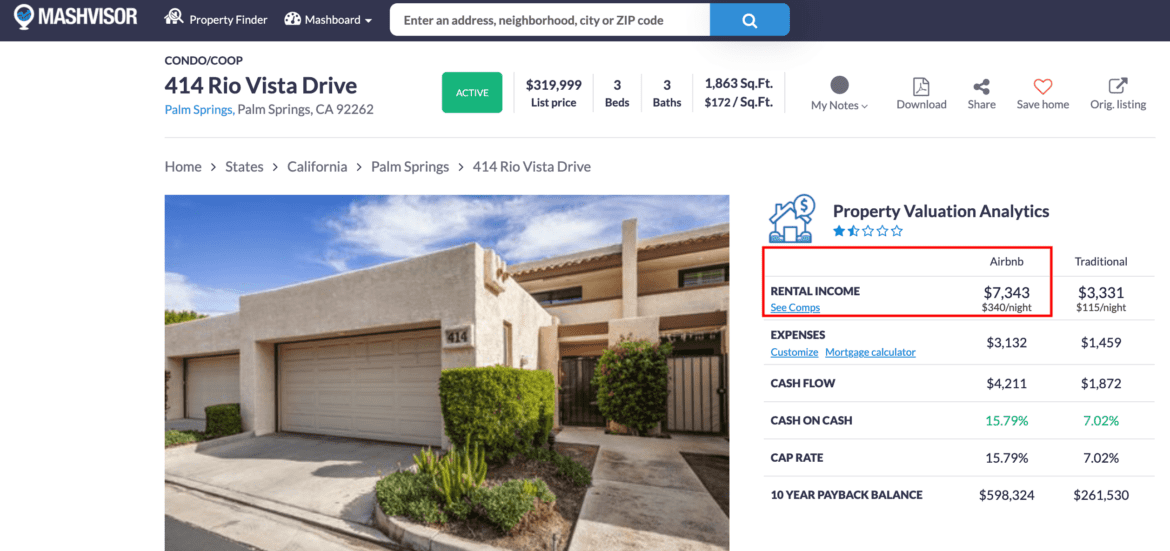**Caption:**

The image showcases a detailed interface of the real estate investment tool, MASHvisor, prominently featuring a property listing. The dark blue top bar includes a search function allowing users to filter by internet address, neighborhood, city, or zip code. The highlighted listing is a condo/co-op located at 414 Rio Vista Drive, Palm Springs, California, 92262. The property is marked 'Active' with a green button, listed at $319,999. It is a 3-bedroom, 3-bathroom residence, spanning 1,863 square feet, priced at $172 per square foot.

Options available for this listing include Notes, Downloads, Share, Saved Home, and Original Listings. Beneath these options, on the left, are details about the home status and address. The photo below this provides a view of a typical beige California stucco building, complete with a garage, a paved walkway, and a gated entrance.

To the right of the property image, MASHvisor’s property valuation and analytics are displayed, comparing different investment options. The metrics include rental income estimates for traditional and Airbnb options, expenses, cash flow, cash on hand percentages, cap rate, and 10-year payback balances. The rental income for Airbnb is projected to be $7,343 per month at a rate of $340 per night, while traditional rentals are estimated at $3,331 per month at $115 per night. This detailed analysis is highlighted within a red rectangle, aiding potential investors in making informed decisions between traditional renting and Airbnb hosting.